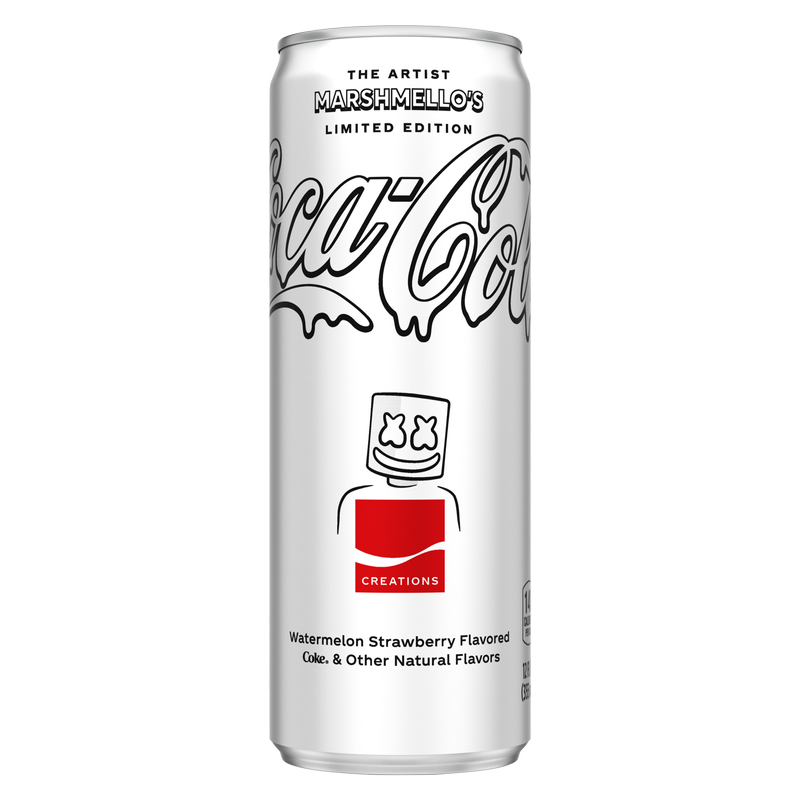The image depicts a tall, cylindrical aluminum Coca-Cola can predominantly white in color, labeled as "The Artist Marshmallows Limited Edition." Starting from the bottom, the can features a flavor description: "watermelon strawberry flavored Coke and other natural flavors." Above this, there is an intriguing illustration of a character with a marshmallow-like head, which possesses two eyes and a banana-shaped smile. This character is donning a white t-shirt that prominently displays a red square on the chest with the word "Creations" inscribed in white within the lower half of the square. Higher up on the can, partially visible is the iconic Coca-Cola branding, showing "CA," the dash, and then "COL." The whimsical design and distinctive elements combine to create an eye-catching and artistic representation of this limited edition beverage.